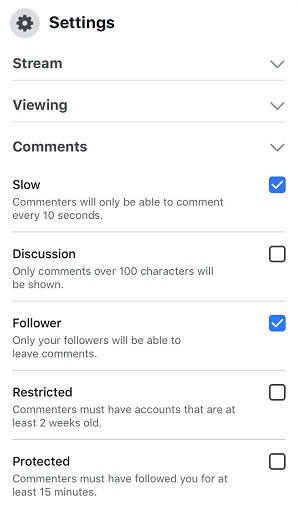**Detailed Caption:**

The image depicts a screenshot of the "Comments" settings within a content creator's streaming application, likely used by a YouTuber or Twitch streamer. The background is a stark white, providing a clean and uncluttered interface. In the upper left corner, there is a gear icon, synonymous with settings menus, accompanied by the bolded title "Settings."

Within this menu, the "Comments" subsection is currently selected, as evidenced by its highlighted state. There are eight specific settings visible, each designed to manage how viewers interact during the live stream.

1. **Slow Mode:** This option is checkmarked, enabling a feature that restricts commenters to posting once every 10 seconds.
2. **Follower-Only Comments:** Also checkmarked, this setting allows only followers of the stream to leave comments, fostering a more controlled environment.
3. **Discussion Mode:** Unchecked, this option, if activated, would allow only comments that exceed 100 characters, encouraging more thoughtful interactions.
4. **Restricted Commenters:** This setting requires commenters to have accounts that are at least two weeks old, a measure likely intended to reduce spam and bot activity.
5. **Protected Mode:** This is another follower-centric feature, wherein only those who have been followers for at least 15 minutes are permitted to comment, ensuring that engagement comes from those with a genuine interest in the stream.

Overall, the settings appear meticulously configured to promote a structured and engaging comment section, enhancing the overall quality of the streaming experience for both the content creator and their audience.